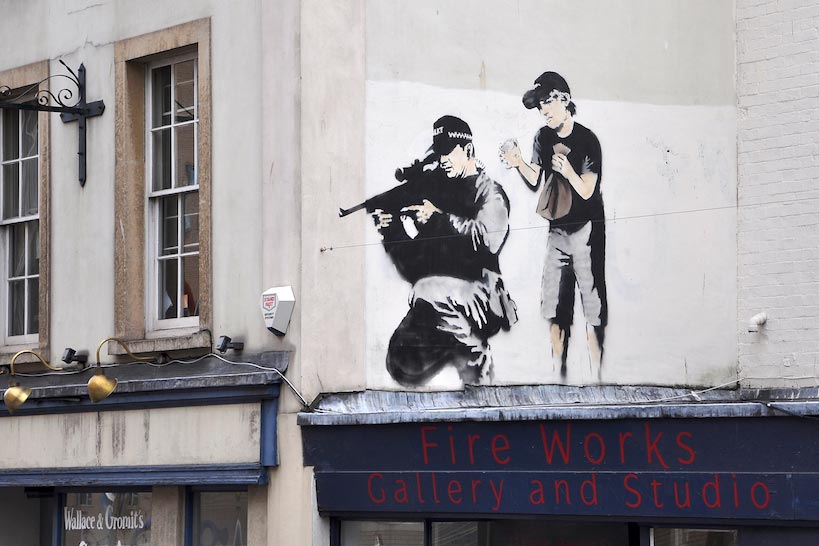This detailed photograph captures a striking mural on the side of a building. The mural, framed within a white square, features a scene reminiscent of Banksy's street art style. To the right of the mural, a brick wall, and to the left, a neighboring two-story stone building with brown stone accents around white-paned windows, frame the artwork. The mural itself depicts a SWAT officer, identifiable by his tactical attire, vest, and a scoped rifle, intently peering through the scope out towards the street. Standing behind him, a little boy in shorts, a black t-shirt, and a black hat mischievously holds a bag in one hand and a cup, or possibly something less discernible, in the other. The dramatic composition extends beyond the mural's white borders, with the rifle barrel and the boy's head breaking through the frame. Below this artwork, a blue awning bearing the inscription "Fireworks Gallery and Studio" adds to the layered urban setting captured in this image.